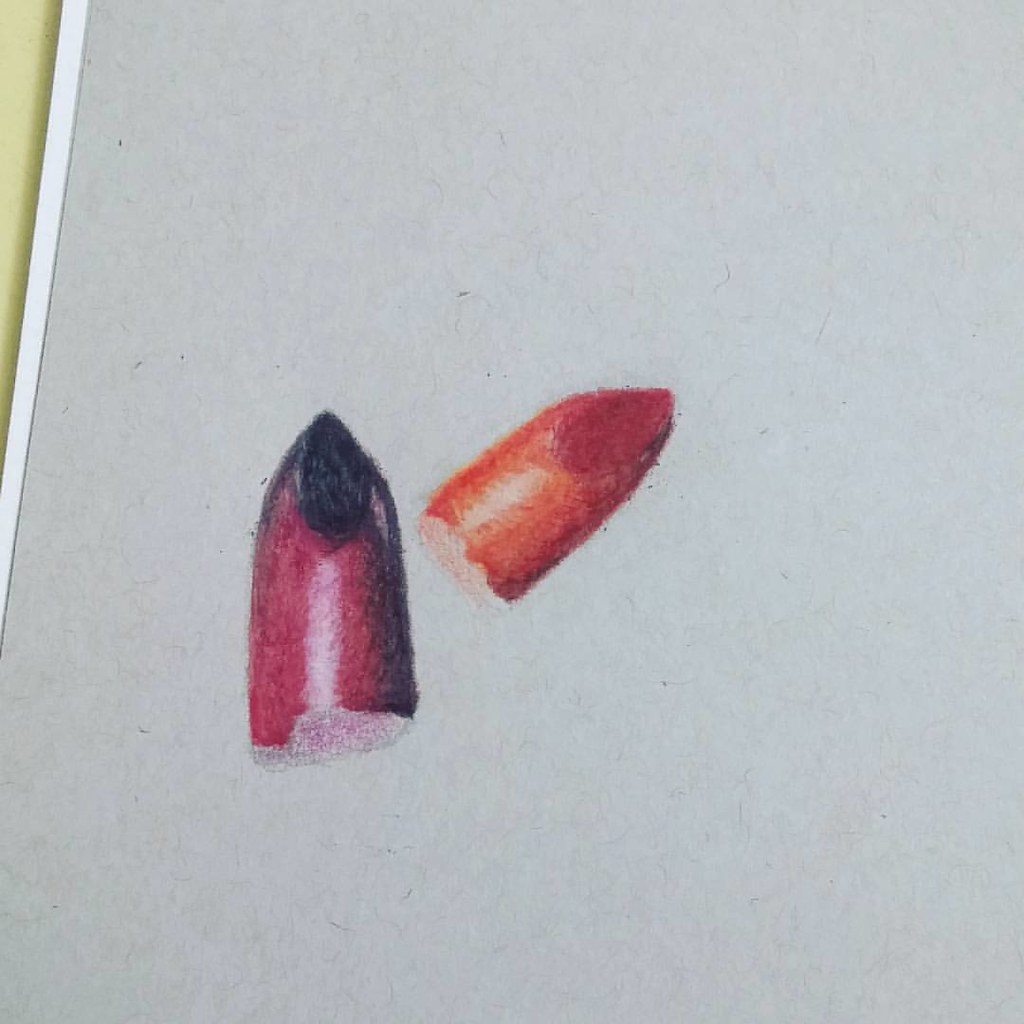This vibrant color photograph showcases a detailed color illustration on a pristine white sheet of paper. The illustration depicts two dislodged lipstick bullets, commonly known as such when detached from their original tubes, which are not shown in the image. The left lipstick bullet is portrayed in a rich purple shade, featuring a jagged edge at its base where it has broken away from the tube. Its tip is distinctly black, adorned with a white vertical line that simulates a reflection or highlight, indicating a light source. Positioned to the right and angled slightly diagonally is the second lipstick bullet, illustrated in a vivid orange hue. Similar to its counterpart, it exhibits a jagged base, signifying its separation from the tube. The tip of this orange bullet is a deeper, darker orange, while the body transitions into a lighter orange shade, creating a striking contrast within the illustration. The meticulous attention to detail in the illustration emphasizes the textures and reflective properties of the lipstick bullets, enhancing the overall depth and realism of the depiction.